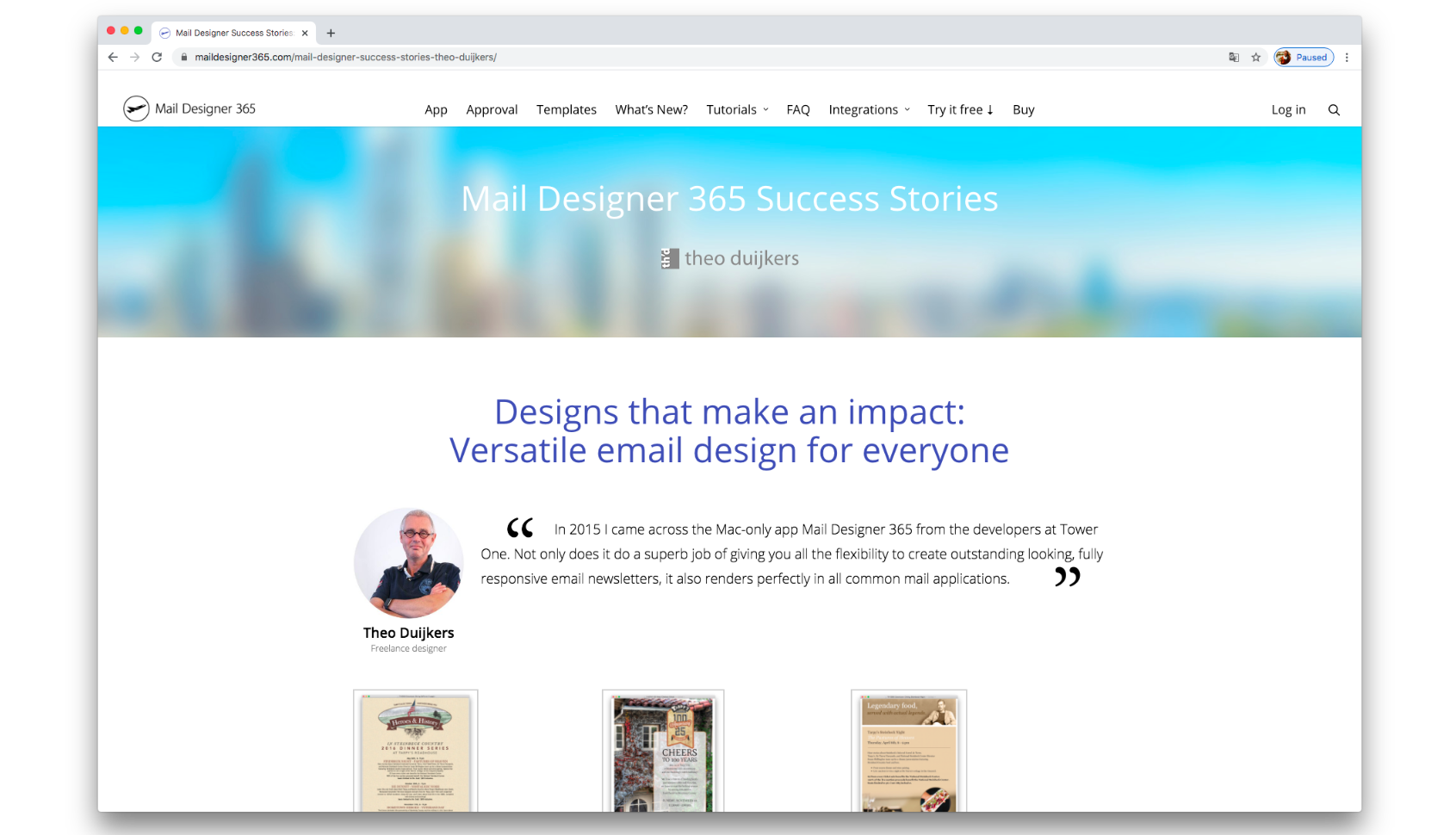This image is a screenshot of the MailDesigner365 website, a platform geared towards email design. The website's name, "maildesigner365.com," is prominently displayed in the top left corner, accompanied by a logo featuring a black circle with an airplane icon ascending diagonally, symbolizing upward progress or takeoff. 

The top navigation bar includes various tabs, listed from left to right as follows: "App," "Approval," "Templates," "What's New," "Tutorials," "FAQ," "Integrations," "Try it Free," and "Buy." Notably, the "Try it Free" tab is marked with a downward-pointing arrow, which is not a drop-down menu but an actual arrow icon.

On the top right of the website, there are user interaction buttons for "Login" and "Search," the latter represented by a magnifying glass icon. Centered at the top of the page is a header titled "MailDesigner365 Success Stories," introducing a section that features testimonials from users. The first testimonial prominently visible is from a user named Theo Dutrix, sharing his positive experience with the platform.